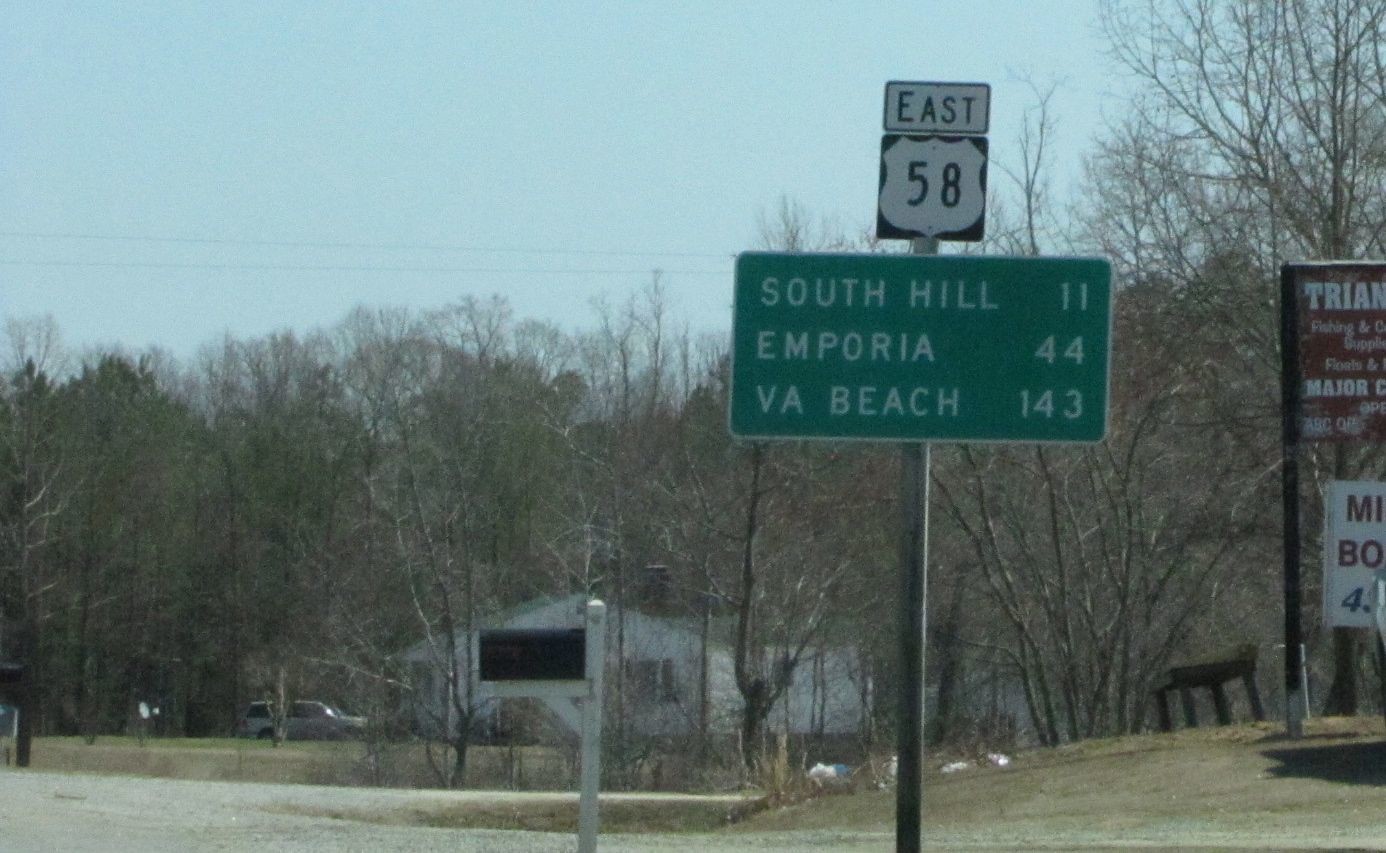The image showcases a series of street signs set against a backdrop of a bluish sky, which appears somewhat muted by a grayish tone. The sky, while clear, suggests the subtle presence of overcast conditions. Scattered across the scene are numerous trees that exhibit minimal foliage, indicative of either autumn or the onset of early spring.

Positioned slightly off-center to the right is a prominent wooden post supporting two key signs. The upper sign, presenting a shield symbol, designates "East 58" for Highway 58. Directly beneath it is a green rectangular sign adorned with white lettering, providing directional distances: "South Hill 11 miles, Emporia 44 miles, VA Beach 143 miles."

In the background, partially shrouded by the leafless trees, stands a white building, adding an architectural element to the otherwise natural scene. Additional signs are partially visible towards the right edge of the photograph, indicating a bustling thoroughfare nearby.